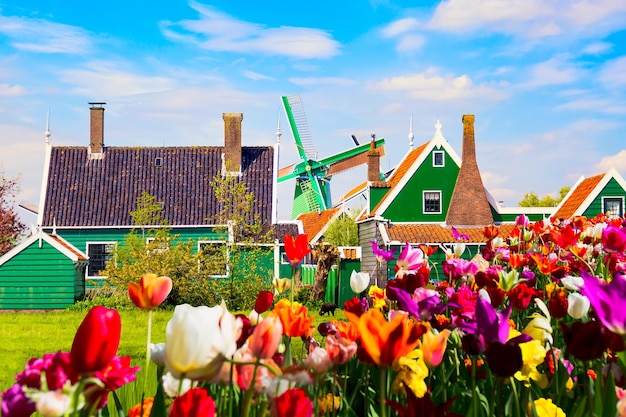A vibrant, detailed painting captures a lush garden of tulips in full bloom, featuring a mesmerizing array of colors: vibrant red and white, red and yellow, purple, orange, and pink. These tulips, some fully open and others just beginning to unfurl, dominate the front foreground. In the midsection stands a pair of picturesque houses. The house on the left is dark green with white-trimmed windows and doors, a steep black tile roof adorned with two tan chimneys. The adjoining house on the right is a brighter green with a red tile roof and a single red chimney. Towering in the center background, a green windmill with four blades adds a quintessentially Dutch charm. This landscape is set against a bright blue sky dotted with scattered clouds, enhancing the picturesque beauty of the scene. The tiny pump house attached could possibly link the two main structures, giving a quaint, united feel to the composition.